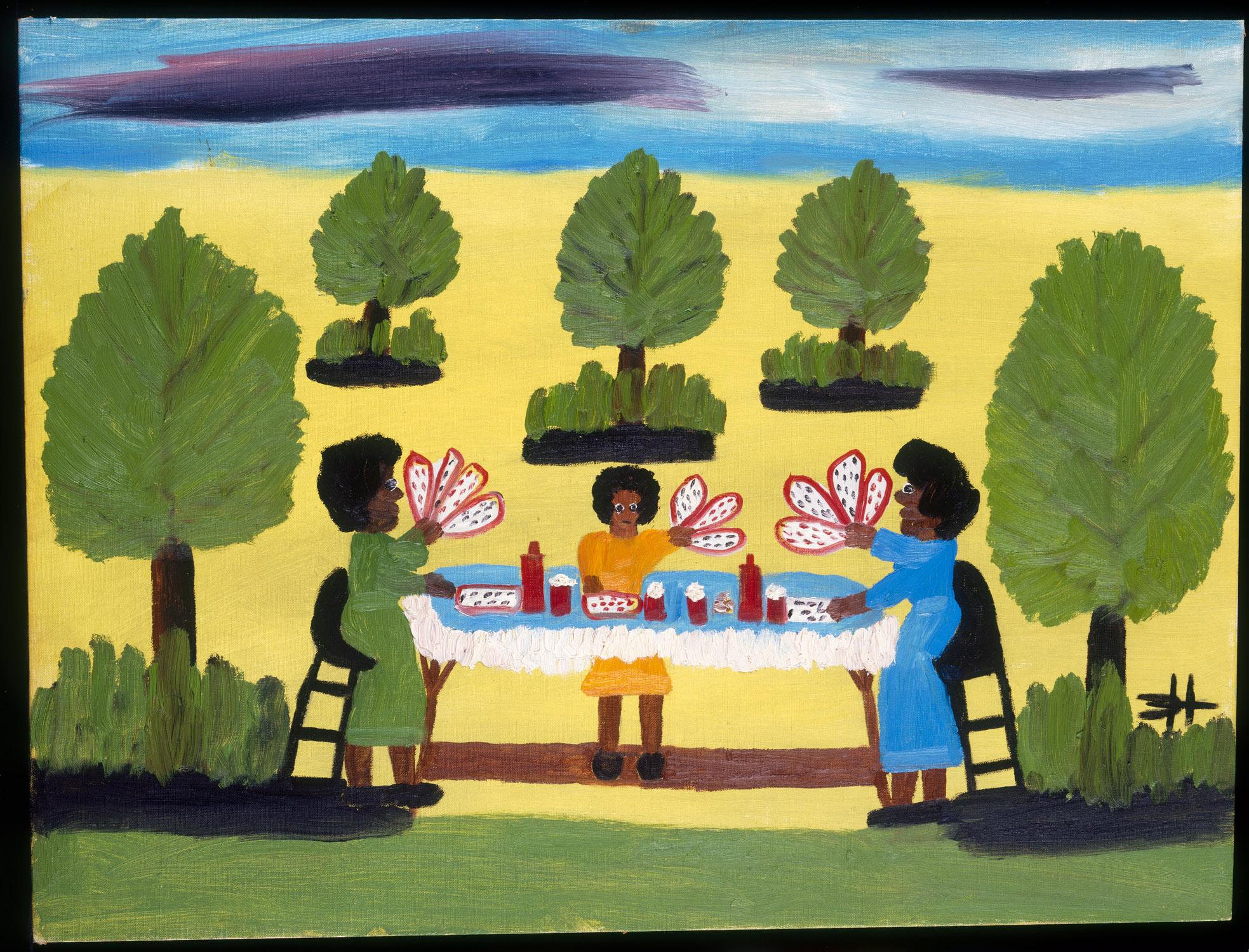The painting depicts a vivid outdoor scene featuring three African-American women seated at a long table covered with a blue cloth. The women, centered in the composition, are engaged in an activity involving red fan-like objects that resemble petals and white, speckled items reminiscent of cactus leaves. Each woman has a distinctive appearance: the one on the left wears a long green dress with black shoes, the middle figure wears an orange dress with black shoes, and the woman on the right dons a blue dress, all with Afro hairstyles.

Behind them, a vibrant background captures the essence of a sunny day with clear blue skies accented by two purple streaks. A strip of yellow and a sliver of green suggest a grassy expanse leading to trees and, possibly, a beach setting. There are five trees in total: two larger ones flanking the scene, and three smaller ones in the distance. 

Red cups and glasses are scattered across the table, hinting at a communal meal or gathering. The use of simple yet bold colors—like the bright blue of the sky, the yellow background, and the green grass—adds a lively and festive atmosphere to the image, suggesting not only a social gathering but also highlighting the distinct African art style.